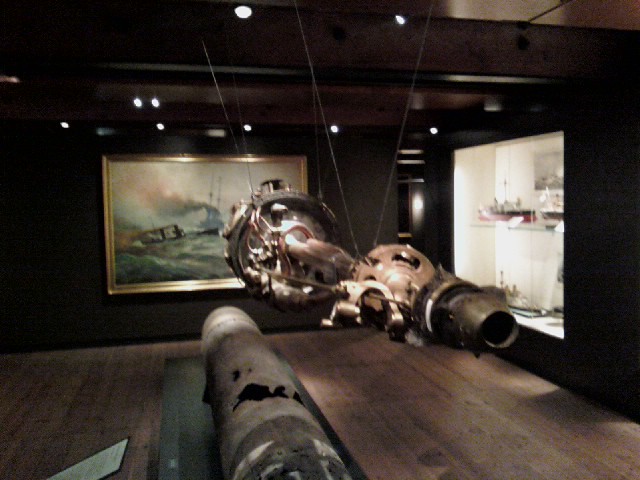The photo captures an exhibit in a museum, prominently featuring a heavy metallic artifact suspended from the ceiling by wires. This mechanical piece, which includes elements resembling a spindle and a gear, is illuminated by ceiling spotlights. Below it, there's a damaged cannon-like object with a significant tear, lying on a green surface next to an unreadable signboard. In the background, a large, gold-framed painting of ships navigating a stormy sea is displayed on the wall. The scene also includes a section on the right with glass windows showcasing designs of large ships and displaying cabinets, all contributing to a rich maritime theme.